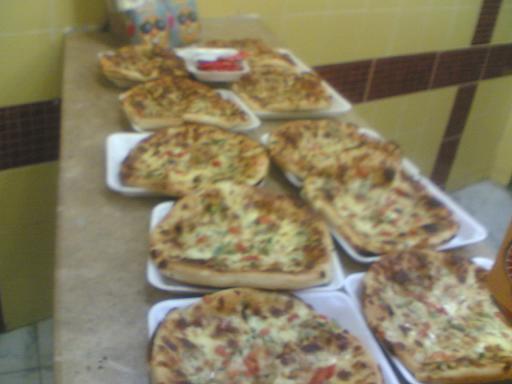In this image, a slightly blurry photograph captures a detailed kitchen or public kitchen scene. The focus is on a countertop stretching diagonally from the bottom right corner towards the top left, though not reaching completely. Adorned with two rows of ten personal-sized, round pizzas placed in neat rows on white square dishes, the dense arrangement has a visually appealing symmetry. Each pizza features a golden-brown crust, browned cheese patches, and a variety of toppings including bright red tomato slices, green herbs, pepperoni, ham, and bacon.

The countertop and dishes are white, while to the right, a white bowl with curled edges contains some unknown red and black items. Against the yellow-tiled wall, which features a striking horizontal and vertical dark brown stripe, sits a carton with two cheerful, sunglass-wearing smiley faces, adding a playful touch to the setting. The balance of colors and arrangement of elements provide a rich, detailed depiction of this lively kitchen countertop.